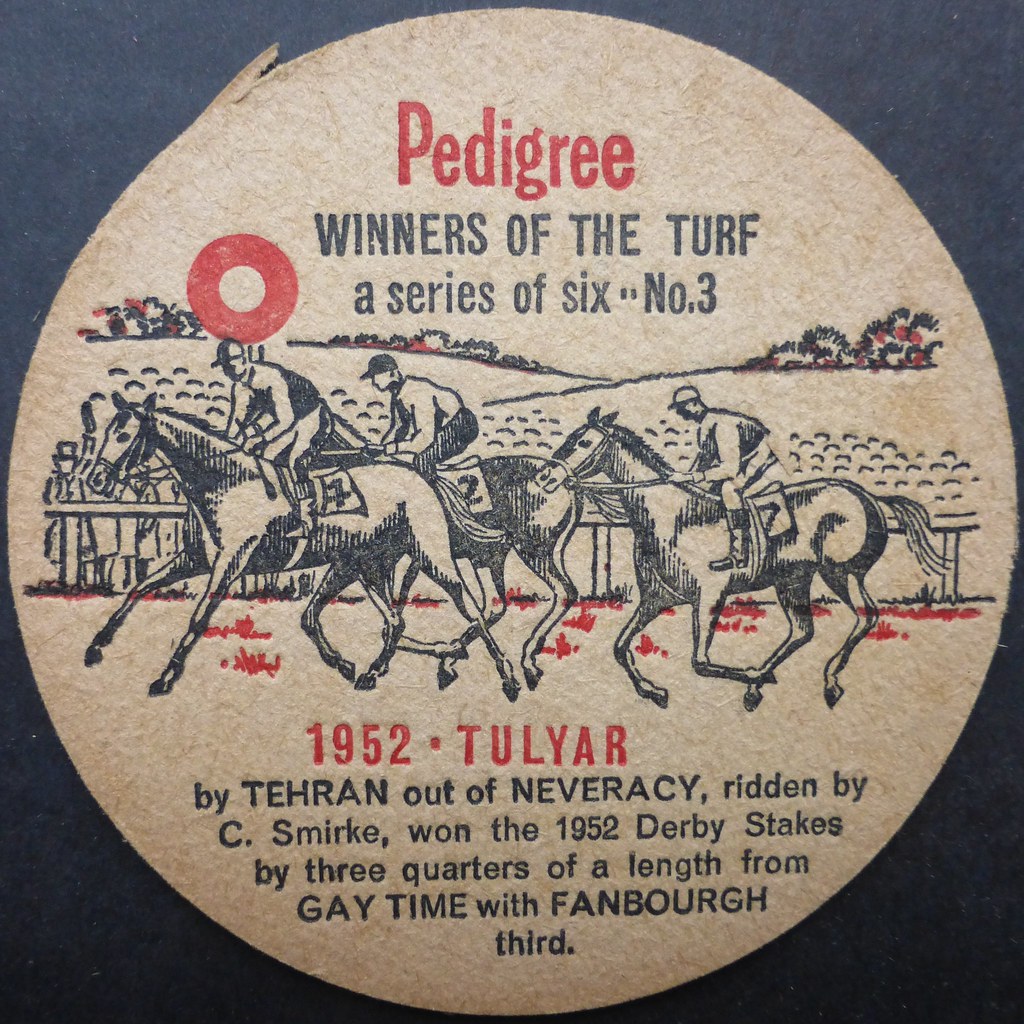This image depicts a round, aged coaster-like object made of cardboard with a light brown, almost beige background and a noticeable rip at the top. Prominently displayed in red at the top, the text reads "Pedigree Winners of the Turf, a series of six, No. 3." Below this title is a detailed black outlined illustration of three jockeys riding horses in a race, with the horses having numbers and a field with a fence and spectators to the left. The grass beneath the horses is depicted in red patches. Further below the illustration, the text in black lettering states, "1952 TULYAR by Tehran out of Neversay, ridden by C. Smirk, won the 1952 Derby Stakes by three-quarters of a length from Gay Time with Fanborough Third." The object appears to be from the year 1952 and could be a collectible item, highlighting its inherent historical and nostalgic value.